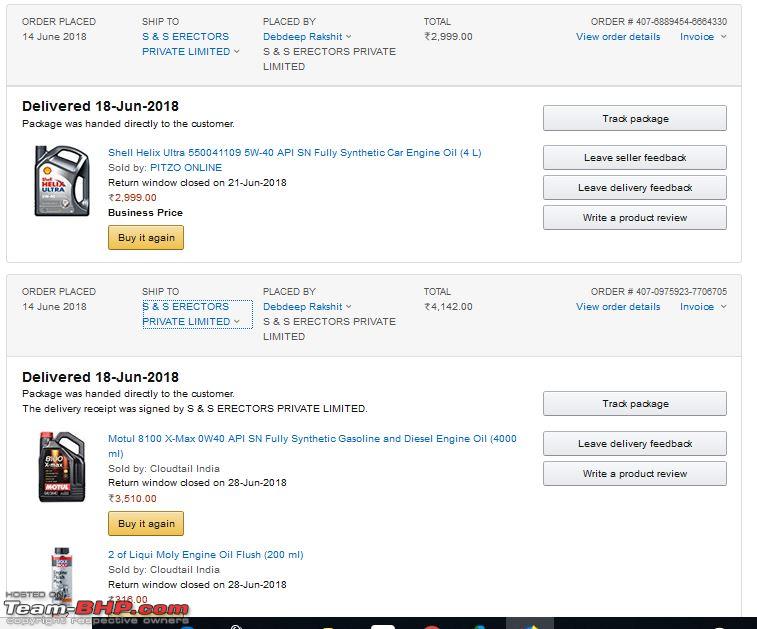The image appears to be a screenshot of an Amazon order status page, detailing multiple items delivered to a customer. In the upper left corner, the order information is displayed, showing that the order was placed on June 14, 2018. The delivery was addressed to "S&S Erectors," and the order was released by "Dead Deep Ratchet." The total order cost amounts to £2,999.

Below this, specific item details are listed:

1. **Item 1:** A bottle of Shell Helix Ultra Fully Synthetic Car Engine Oil, priced at £2,999. This item was delivered on June 18, 2018, and the return window has closed.

2. **Item 2:** Another delivery, received on June 18, 2018, includes synthetic gasoline diesel engine fuel.

3. **Item 3:** Two units of Liqui Moly Engine Oil Flush, also delivered on June 18, 2018.

Each item is accompanied by its respective delivery date and return status, providing a clear and comprehensive overview of the order fulfillment.